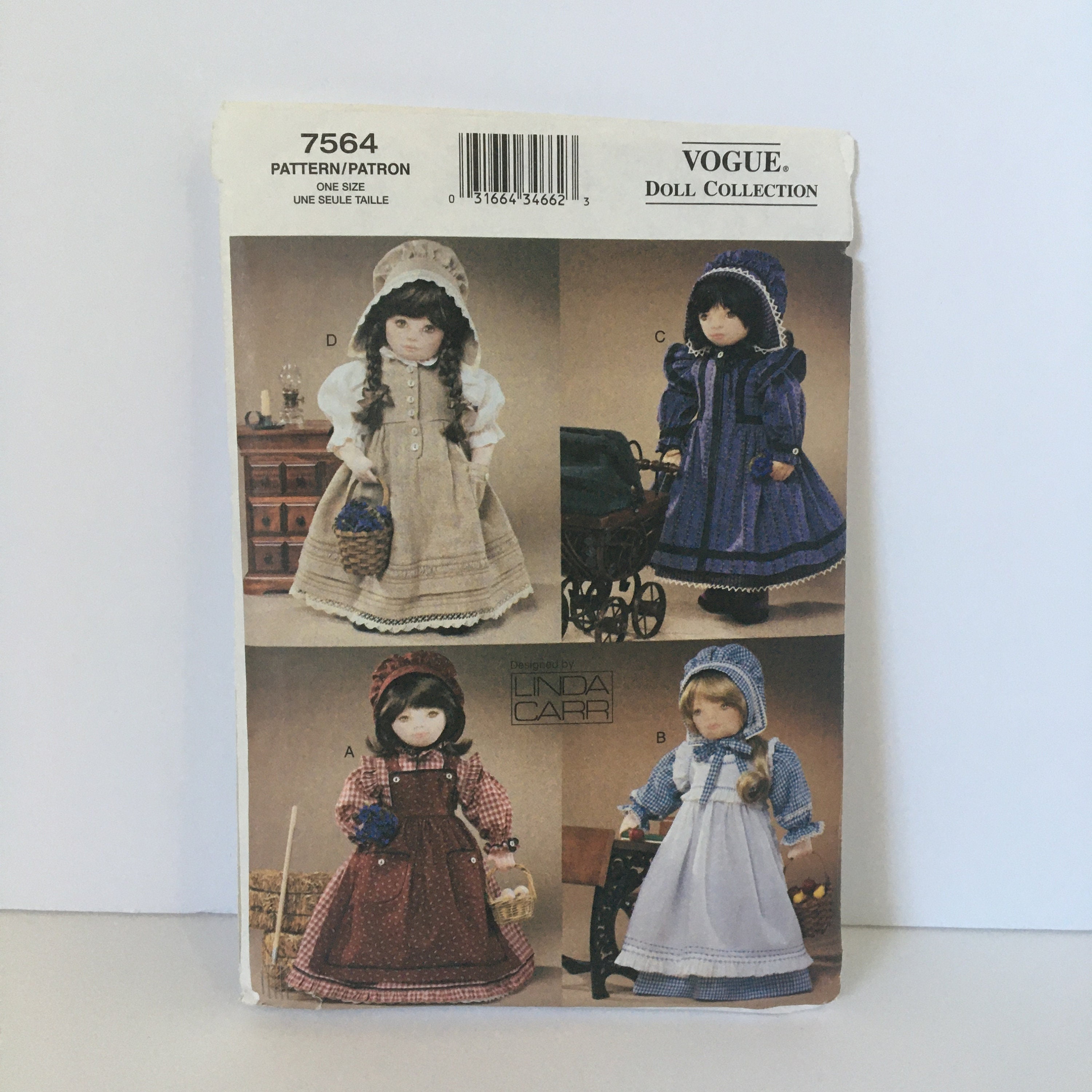This image depicts a vintage advertisement for the Vogue Doll Collection, pattern number 7564. The scene is set against a light cream-colored backdrop that appears to be an upright cardboard stand with slight tears visible on the bottom left and upper right corners. The top left features the text "7564" in black, signifying the pattern number, alongside the words "Pattern, One Size." Prominently positioned at the top is the title "Vogue Doll Collection," and a barcode can be seen in the top middle area.

The advertisement showcases four distinct dolls, each labeled from A to D, clothed in period attire and positioned in individual quadrants. Doll 'A' is adorned in a vibrant red dress with matching bonnet, exuding a classic farm girl charm. Doll 'B' wears a white dress accented with blue plaid and a blue bonnet, giving off a country aesthetic. Doll 'C' sports a Victorian-inspired blue dress with a matching bonnet, and is positioned beside a black baby carriage. Finally, Doll 'D' is dressed in a long beige dress with white sleeves, holding a basket with a blue item, her hair styled in long braids. She stands next to a dresser bearing a candle and a kerosene lamp, enhancing the vintage ambiance of the scene.

Each doll is meticulously detailed, contributing to the overall nostalgic and collectible appeal of this Vogue Doll Collection advertisement.